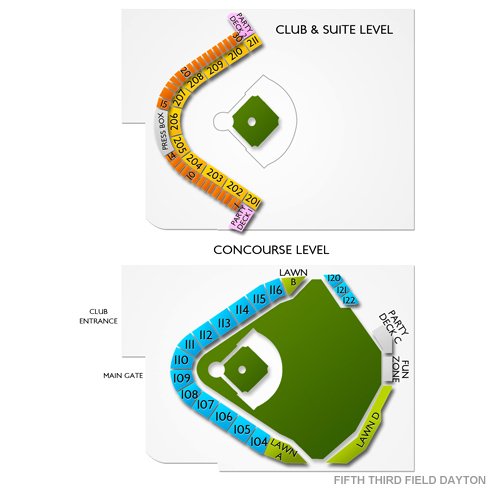This detailed seat map of Fifth Third Field in Dayton is divided into two main sections: the Club and Suite Level, and the Concourse Level. 

At the Club and Suite Level, the map identifies sections in the 200 and 300 ranges. Sections 200 are highlighted in yellow, while the higher tier 300 sections are not specifically color-coded. A special Party Deck is marked in orange, with an adjacent press box indicated in white. The playing field, depicted in green, is surrounded by white sections that likely represent the stadium's infrastructure.

The Concourse Level map features a more expansive view of the field of play, still colored green. Lawn sections are designated with letters (A, B, and D) and shown in green, while the main 100 seating sections are highlighted in blue. Important visitor areas like the Party Deck and the Fun Zone are marked in white. Key access points including the Club Entrance and the Main Gate are clearly labeled on the left-hand side in black text.

The bottom of the map prominently displays the stadium's name, "Fifth Third Field Dayton," confirming the location. While the precise sport isn't explicitly mentioned, visual cues such as the shape of the playing field strongly suggest it is a baseball stadium.